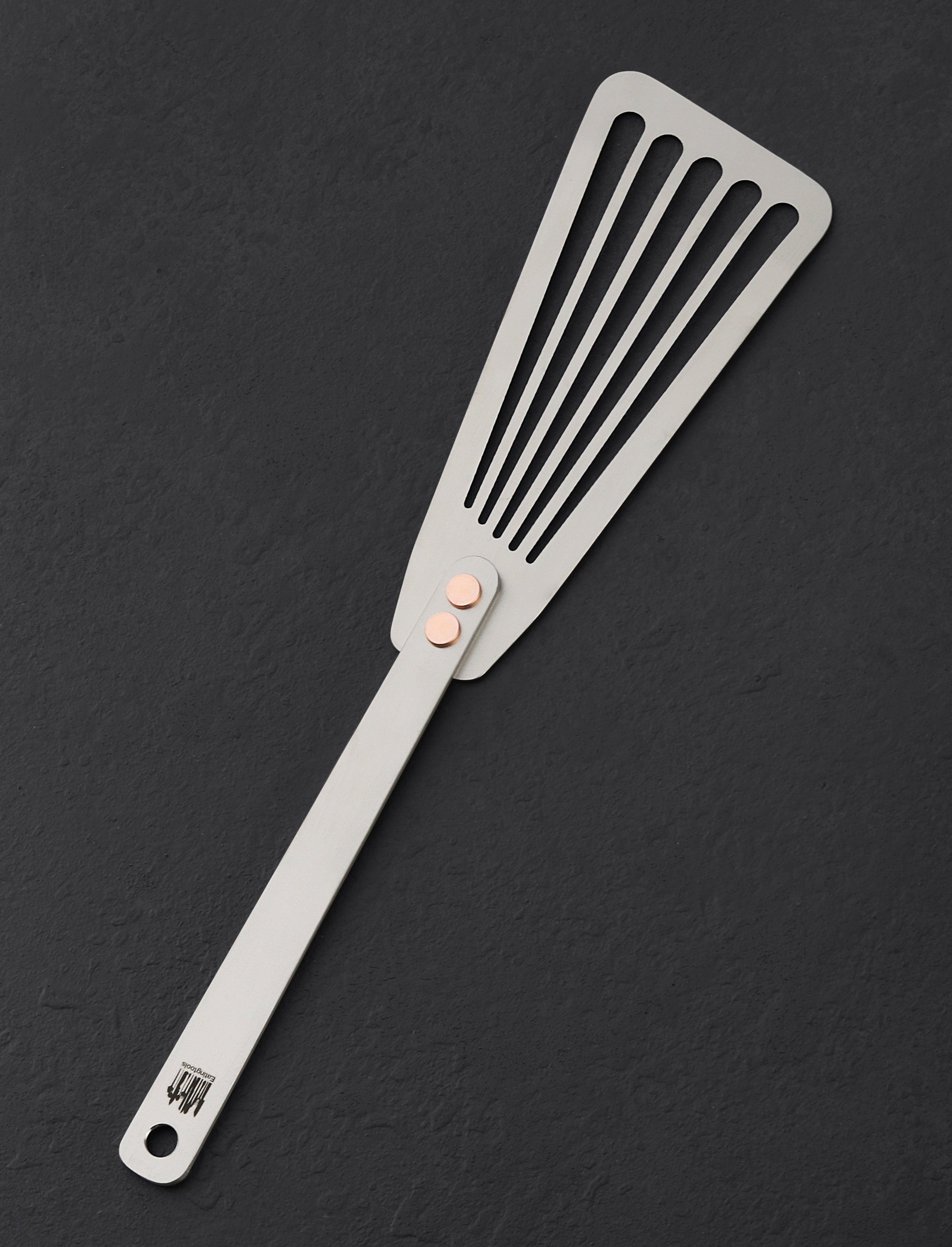This image features a brand-new stainless steel spatula positioned diagonally from the bottom left, where the handle resides, to the top right, where the spatula part is, on a dark gray textured background. The spatula's slim, silver design includes a handle affixed to the main flat metal surface with two brass-colored, welded nails. It is a long utensil designed for cooking, with five slits along the broad part of the spatula to make it easy to lift food from a pan while allowing grease to drip through. The handle, while not particularly ergonomic and more block-cut in style, culminates in a hole for hanging. There is a logo on the handle that is not legible from this angle. The overall aesthetic and functional design suggest it would be highly effective for grilling, effortlessly scraping off food residue while maintaining the integrity of the food.